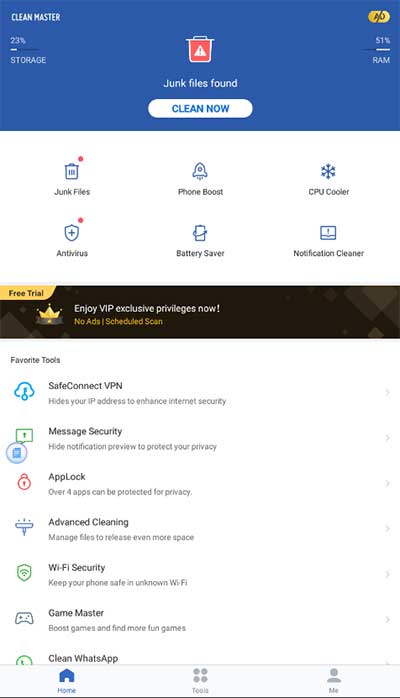Screenshot of a cell phone interface displaying the app "Clean Master." The image features a blue bar at the top with "Clean Master" written in white text on the upper left, alongside the number "23%". Below this, there's a white line partially filled with a darker blue indicating storage usage, and the word "Storage" written in white beneath it.

Prominently in the center is a red trash can icon with a red exclamation mark inside a white triangle, accompanied by the text "Junk Files Found." Below this is a white button with "Clean Now" written on it. 

In the upper right corner, a logo in a bluish-yellowish hue displays "51%" with the word "RAM" underneath, indicating the amount of RAM currently in use. 

The background of the interface is white and features a 3 by 2 grid of functional icons:
1. **Junk Files** with a trash can icon.
2. **Phone Boost** with a rocket icon.
3. **CPU Cooler** with a snowflake icon.
4. **Antivirus** with a shield icon.
5. **Battery Saver** with a battery icon.
6. **Notification Cleaner** with an open book icon.

Both the Junk Files and Antivirus icons have a red dot in their upper right corners.

At the bottom of the screenshot, there's an ad with a black background. In the upper right of the ad is a yellow square with "Free Trial" written in black. The ad itself is promoting a "Safety Connect VIP" package and lists features such as Message Security, App Lock, Advanced Cleaning, Wi-Fi Security, Game Master, and Clean WhatsApp. Additionally, the tab bar at the bottom displays options labeled "Home," "Tools," and "Me."